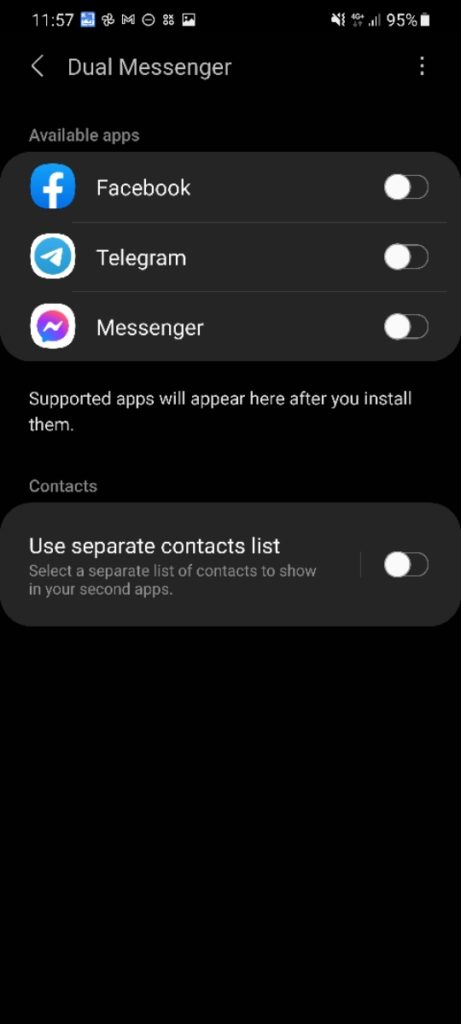Screenshot of the "Dual Messenger" screen on a mobile device. The screen is predominantly black with white text, listing available apps—Facebook, Telegram, and Messenger—all of which have their toggle buttons switched off. Below the list, a message indicates that supported apps will appear after installation. There is an additional toggle for "Use Separate Contact List," which is also off. The screen shows the icons for Facebook, Messenger, and Telegram. A small battery icon at the top right corner indicates 95% battery life. The clear white text contrasts sharply against the dark background, ensuring readability.